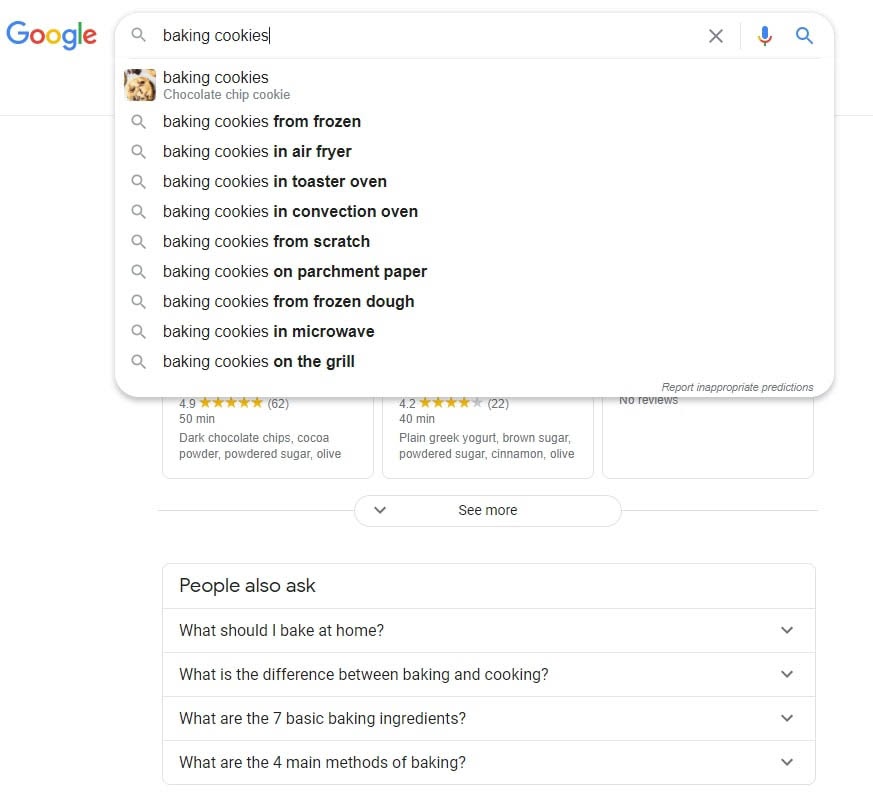The screenshot captures a Google search interface on a desktop, showcasing the familiar layout against a clean, white background. On the left side, the vibrant, multicolored Google logo stands out, while on the right, the prominent search box is displayed.

Within the search box, the query "baking cookies" is typed in black text, accompanied by a gray search icon. Included alongside are an 'X' button to clear the input, a microphone icon for voice search, and a blue search button to initiate the search.

The dropdown beneath the search box presents several instant search suggestions. It starts with "baking cookies" and an icon of cookies, followed by various other related search prompts such as "baking cookies from frozen," "baking cookies in air fryer," "baking cookies in the toaster oven," "in convection oven," "from scratch," "on parchment paper," "from frozen cookie dough," "in microwave," and "on the grill."

Partially visible behind the dropdown menu are user reviews for different recipes, with ratings of 4.9 stars and 4.2 stars, respectively. Below these, a "See more" box with an arrow suggests further content.

Further down, five segmented boxes come into view, starting with "People also ask" in bold. These segments include frequently asked questions such as "What should I bake at home?" with a dropdown arrow, "What is the difference between baking and cooking?" with another dropdown arrow, "What are the seven basic baking ingredients?" with an additional dropdown arrow, and finally, "What are the four main methods of baking?" also with a dropdown arrow.